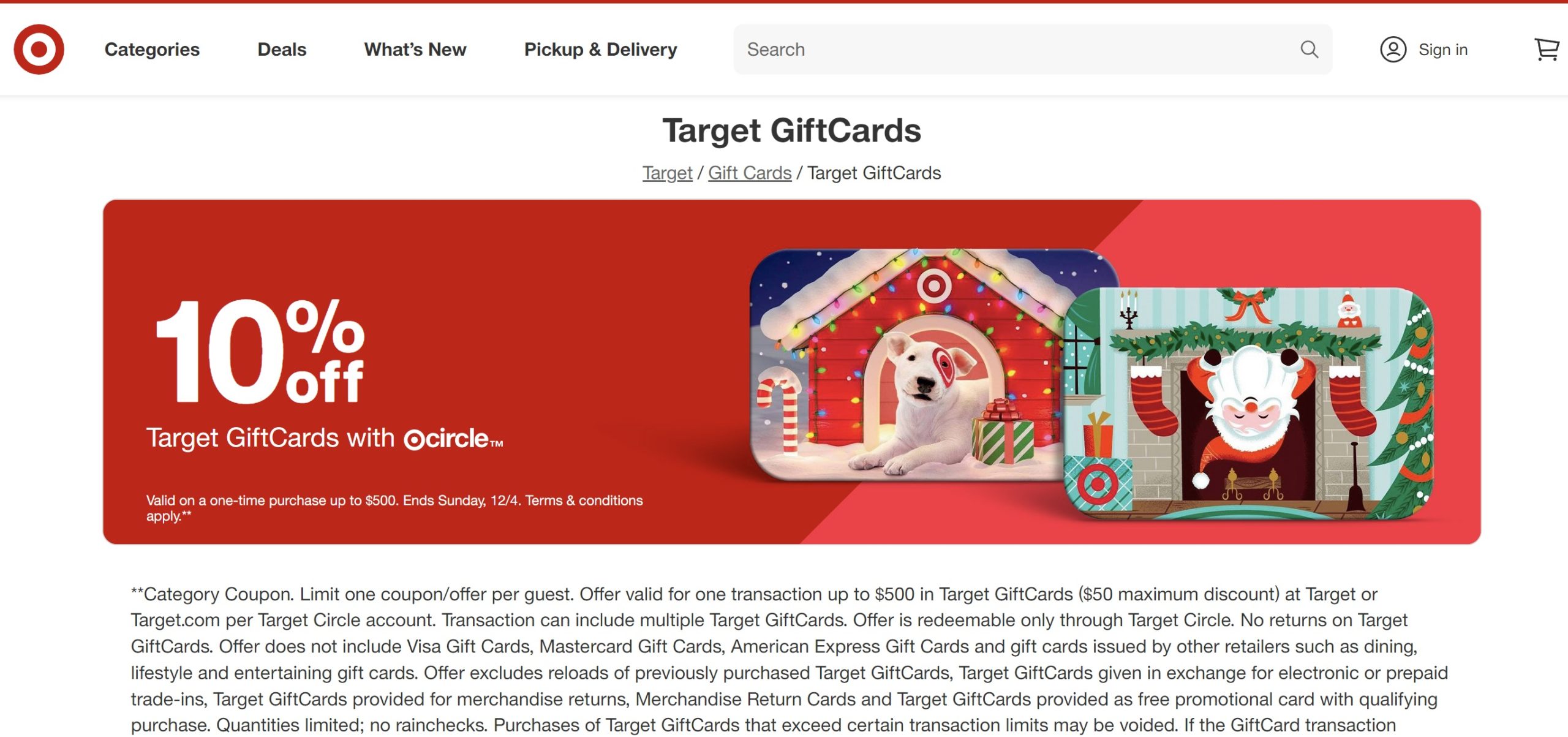The image is a horizontal rectangle with the longer side running from left to right. At the very top is a thin red line stretching across the entire length of the image. Directly below this line, on the left side, is the iconic bullseye logo for the company Target. Moving rightward from the logo, there is a navigation menu with the following options in black text: "Categories," "Deals," "What's New," and "Pickup & Delivery." Adjacent to these options is a shaded gray search box featuring a magnifying glass icon, representing the search function. Further to the right, there is a sign-in area and a shopping cart icon. A very faint gray line runs beneath this top section, demarcating it from the rest of the image.

Below this line, the text "Target Gift Cards, Target Gift Card, Target Gift Cards" appears prominently. Beneath this text is a large red rectangle. On the left side of this rectangle, white text reads "10% off Target Gift Cards with Circle," accompanied by a smaller blurb in a tiny font. Within the red rectangle, two holiday-themed Target gift cards are displayed. One card features a dog sitting in a festively decorated doghouse, while the other card shows Santa Claus descending through a chimney. Below these gift cards is a paragraph likely detailing the terms and conditions associated with the gift card promotion.